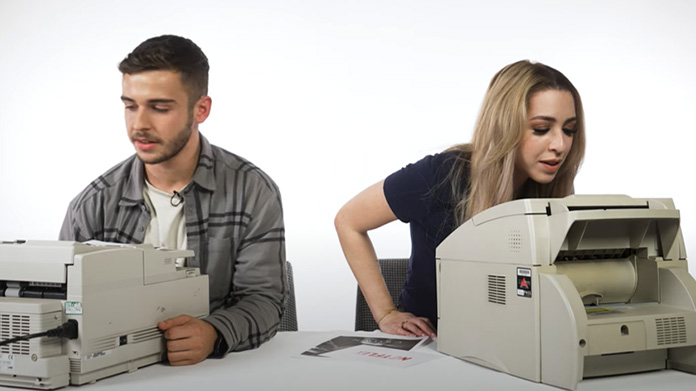In the photograph, two Caucasian individuals are positioned side by side in front of two copy machines, against a white wall. The man on the left, who has short brown hair, a mustache, and a goatee, is dressed in a white t-shirt layered with an open gray and black flannel shirt. He rests his hand on the side of his copy machine, which is plugged in with a visible black plug. His machine bears a black and red label on the side. The woman on the right, with long blonde hair, is seated in a black chair and leans slightly forward while focusing intently on her own copy machine. She is dressed in a dark blue shirt and wears a ring on her middle finger. There is a printed piece of paper on the desk between them, and the desk itself is long and gray. Additionally, a small sign with red lettering is visible near the woman's equipment. Both individuals appear to be engaging with tasks related to the machines, although the woman's concentration is more evident than the man's.